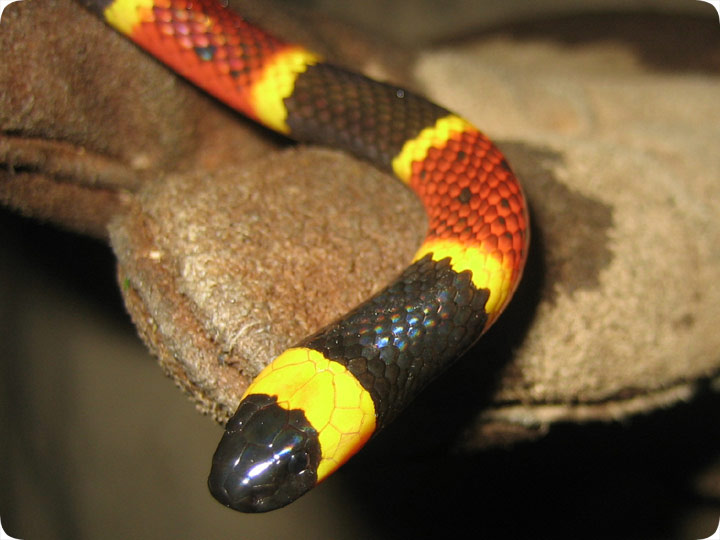This is a close-up color photograph of a slender snake, possibly a coral snake, showcasing its distinctive pattern of black, yellow, and red rings. The snake has a shiny black head, followed by alternating bands of yellow, black, yellow, orange-red, and yellow again. The pattern repeats in the sequence: yellow, black, yellow, red-orange, yellow, black. Its vibrant scales glisten in the light, particularly where the black bands are prominent. The snake's eye is clearly visible, peeping off the side of a stone that is brown and may be surrounded by a pair of gloves or a leather-like textured surface with wrinkle details, indicating a close-up. The reptile appears to be slithering or coiled on this surface, which could be a worn piece of cloth or leather. The backdrop is mostly brownish, possibly indicating a natural setting, and there might be water in the background. There are no humans or text in the image, focusing solely on the snake as it peeks off the edge of the rock-like surface.